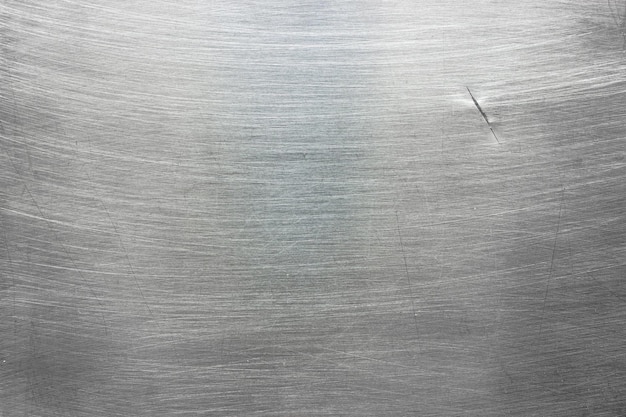The image depicts a close-up of a well-used stainless steel surface, likely a metal prep table or a piece of industrial equipment. The metal is predominantly silver, adorned with numerous scratches that vary in direction, with many running horizontally from left to right. These scratch marks suggest both heavy use and extensive cleaning over time. A noticeable feature is a cut or slash near the upper right corner, revealing a darker background within the split, which contrasts sharply with the shiny, reflective surface of the metal. The lighting highlights some areas, giving the surface a darker appearance in spots. The overall image captures the texture and wear of the metal, conveying a sense of its utilitarian purpose.